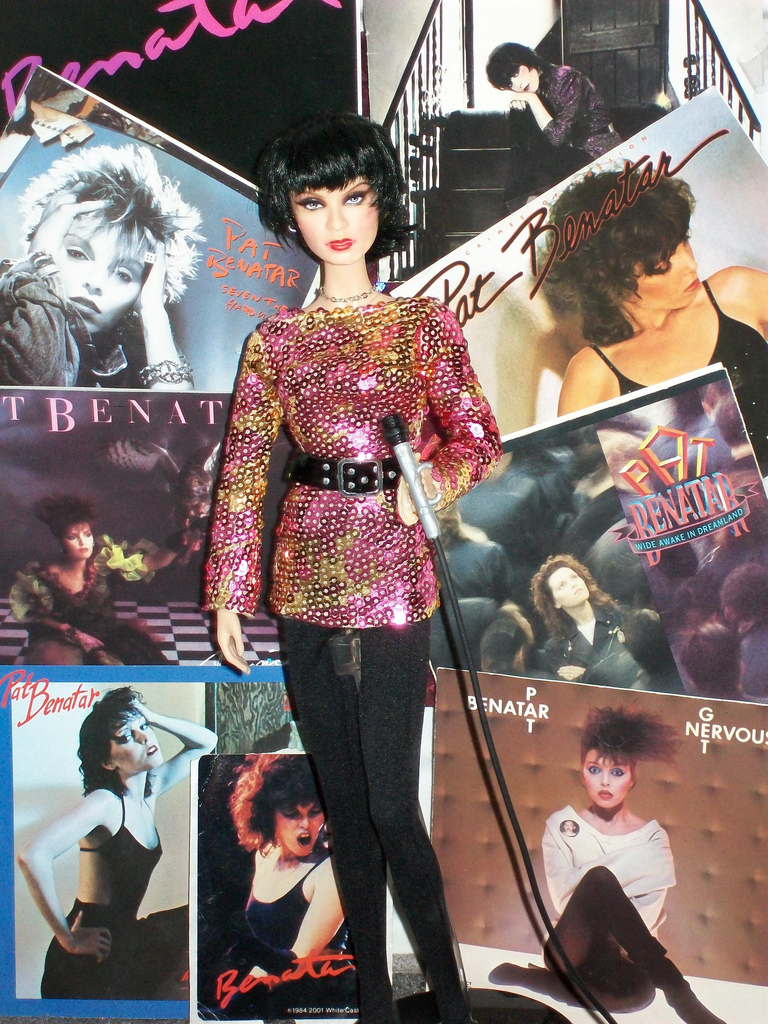This photo showcases a doll designed to resemble the iconic singer Pat Benatar, standing in front of a backdrop that prominently features a collage of her album covers. The doll is dressed in black pants paired with a sequined, multi-colored dress shirt that transitions from red to yellow. Highlighting the ensemble is a black belt cinching the shirt at the waist. The doll's short black hair, red lipstick, and eyeshadow add to its striking appearance. Around its neck, it wears a silver chain necklace, and in its left hand, positioned on the right side of the image, it holds a silver and black plastic microphone with a cord trailing off-screen. The stage-like setup and attention to detail in the outfit and accessories suggest a tribute to Pat Benatar, with numerous album covers, including one depicting her in a padded room, visible in the background.